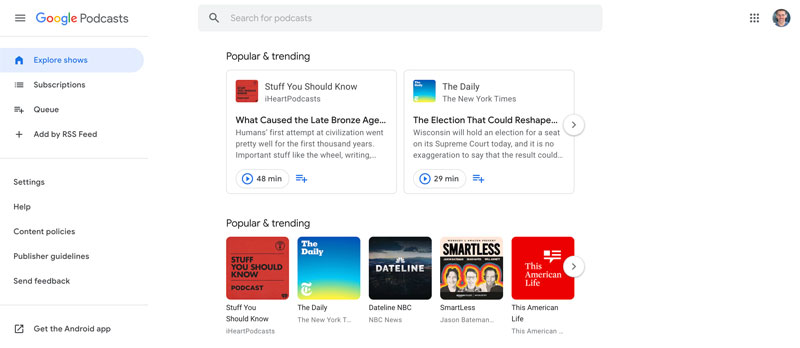The screenshot captures a detailed view of the Google Podcasts web page. On the left side, there's a column of navigation options beginning with a symbol of three horizontal lines, the colorful Google brand logo, and the gray text, "Podcasts." A gray dividing line separates this header from the selected option below, "Explore Shows," which features a blue house icon within a light blue rounded box, indicating it is currently active. Additional navigation options are listed in black, indicating they are not selected: "Subscriptions," "Queue" (with a plus symbol), and "Add by RSS Feed." Another gray dividing line follows, separating from further options like "Settings," "Help," "Content Policies," "Publisher Guidelines," and "Send Feedback." Below, an icon of a box with an arrow pointing upwards and the text "Get Android App" appears. 

To the right, the main content area displays search results. At the top, a gray search bar features a magnifying glass icon and the placeholder text "Search for Podcasts." Below, the "Popular and Trending" section showcases two podcasts: "Stuff You Should Know" from iHeart Podcasts with its latest episode titled "What Caused the Late Bronze Age," lasting 48 minutes, and "The Daily" from the New York Times with the episode "The Election That Could Reshape..." about Wisconsin, lasting 29 minutes. Each entry includes a brief description and a blue play button.

Further down, additional entries for the "Popular and Trending" section are depicted in a grid layout, featuring thumbnails for "Stuff You Should Know," "The Daily," "Dateline NBC," "SmartLess," and "This American Life." In the far upper right, the interface shows a 3x3 grid of squares alongside a Google profile avatar of a middle-aged white man.